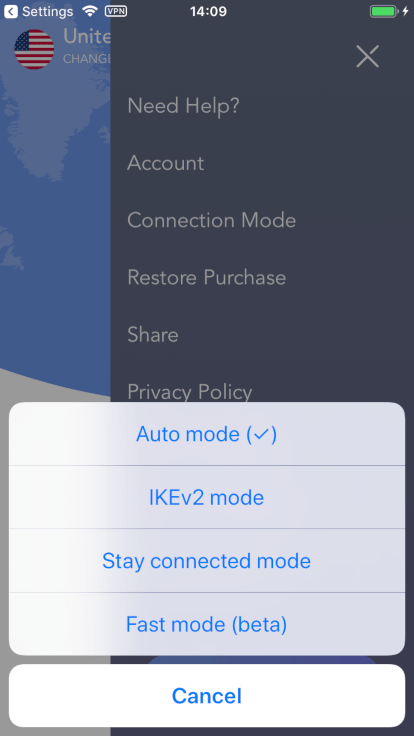A detailed and cleaned-up caption for the described image could read:

"Screenshot of a cell phone's settings page with an active pop-up overlay. The phone's wallpaper features a stylized map of the world in shades of gray and blue. In the status bar at the top, white icons indicate active settings, Wi-Fi, and VPN connections. The time, displayed in the center, reads 14:09, while the battery icon on the right shows almost full capacity, marked by a green bar and a lightning bolt. 

The home screen includes an icon of the U.S. flag with red, white, and blue stripes and a section of the blue field with white stars. Layered on top is a semi-transparent charcoal gray pop-up with an 'X' in the upper right corner to close it. This overlay lists categories such as 'Need Help,' 'Account,' 'Connection Mode,' 'Restore Purchase,' 'Share,' and 'Privacy Policy.'

Within the pop-up, four selectable options in blue font are divided by light gray lines: 'Auto Mode' with a check mark in parentheses, 'IKEV2 Mode,' 'Stay Connected Mode,' and 'Fast Mode (Beta).' At the bottom of this list lies a white pill-shaped button labeled 'Cancel.'"